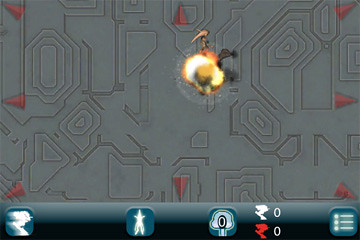This image portrays a video game interface featuring a dark gray background with intricate black maze-like lines distributed across the screen. Prominently placed in each corner and the center of each side are striking red triangles. At the top center of the frame, there is a vivid fireball explosion with visible flames and debris. The bottom section of the screen displays a series of five icons. In the bottom right corner, there is a hamburger menu icon. To the left of this menu, a scoreboard displays the score as "00." Additional icons to the left allow for further interaction and progression within the game.